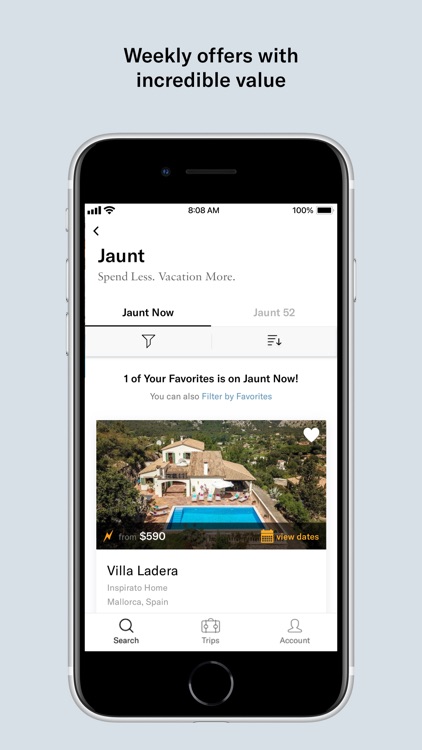A pale blue-gray background hosts a detailed promotional ad. A cell phone displays a booking app interface, complete with visible buttons along its sides and bottom. The screen showcases various details: 

- At the top, black text reads, "Weekend Offers with Incredible Value."
- Beneath this header, the phone's status bar indicates the time as 8:08 a.m. and shows a fully charged battery at 100%.

The app's interface presents:
- A left arrow followed by text on the left stating, "Jaunt - Spend Less, Vacation More."
- Tabs for navigation: "Jaunt Now," "Jaunt 52," with "Jaunt Now" currently selected.
  
Further down:
- Icons for a filter option and sorting function (displayed as descending lines with an arrow).
- A section header that reads, "One of Your Favorites is on Jaunt Now. You can also filter by Favorites," highlighted in blue.

Below the filter section:
- A photograph showcases a luxurious backyard featuring an expansive blue pool.
- Overlay text indicates, "590 View Dates," accompanied by a white heart icon filled in, signifying a favorite.

Adjacent details include:
- The property is identified as "Villa Ladera, Inspirational Home, Mallorca, Spain."

At the bottom of the display:
- Navigation icons for "Search" (with a magnifying glass), "Trips" (with a suitcase), and "Account" (with a person icon).

This detailed image offers a glimpse into a travel app promoting exclusive vacation deals.